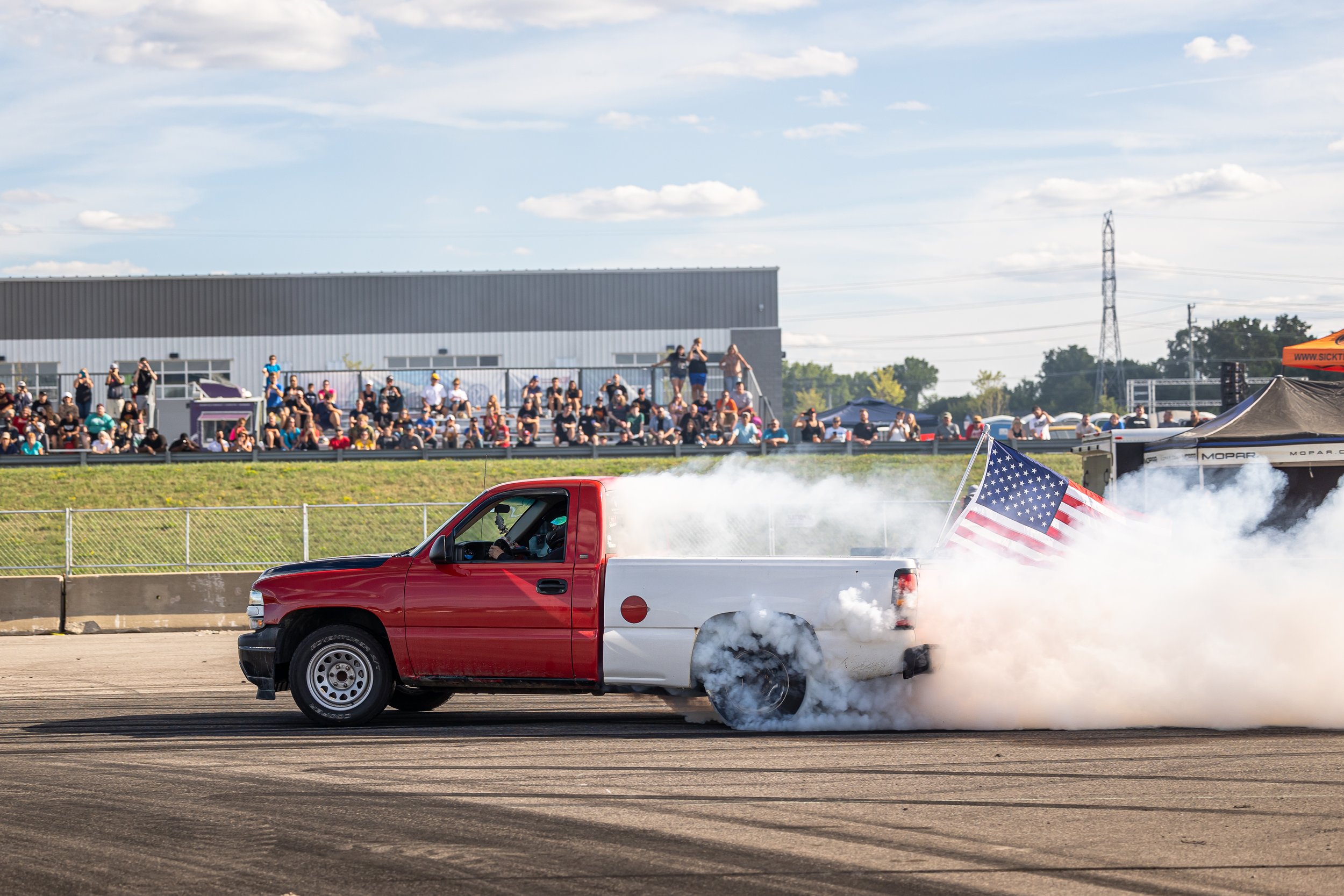In this vibrant and dynamic daytime photograph, a red and white pickup truck is prominently featured as it drives counterclockwise on a dirt track. The truck, with its red front half and white-painted bed, spins its wheels energetically, producing a thick bar of whitish-gray smoke that billows out from behind the cab, obscuring parts of the scene. Attached to the back of the truck bed is an American flag, partially veiled by the swirling smoke.

A crowd of spectators can be seen gathered on a green hillside and standing behind a fence, intently observing the action on the track. They are a mix of onlookers, some sitting on benches and others perched on shoulders, all engaged with the spectacle before them. The sky above is a mix of blue and clouds, adding to the lively and bustling atmosphere of what appears to be a track race or truck rally event. The overall scene is filled with enthusiastic energy, with the audience cheering and capturing the thrilling moment.